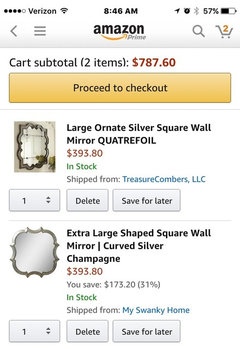Screenshot from a phone displaying the Amazon shopping cart page. The phone is on Verizon service with a full signal and the battery is at 57%. The Amazon logo features its iconic yellow arrow curving under the bottom. The shopping cart shows two items with a subtotal of $787.60. A yellow-orange "Proceed to checkout" button is visible beneath the subtotal.

The first item in the cart is a "Large Ornate Silver Square Wall Mirror, Quadrafoil," priced at $393.80. It is in stock and shipped from Treasure Commerce, LLC. Quantity: 1. 

The second item is an "Extra Large Shaped Square Wall Mirror, Curved Silver Champagne," also priced at $393.80, originally $567.00, providing a savings of $173.20 (31%). This item is in stock and shipped from My Swanky Home. Quantity: 1.

In summary, the cart holds two mirrors with detailed descriptions and savings information.